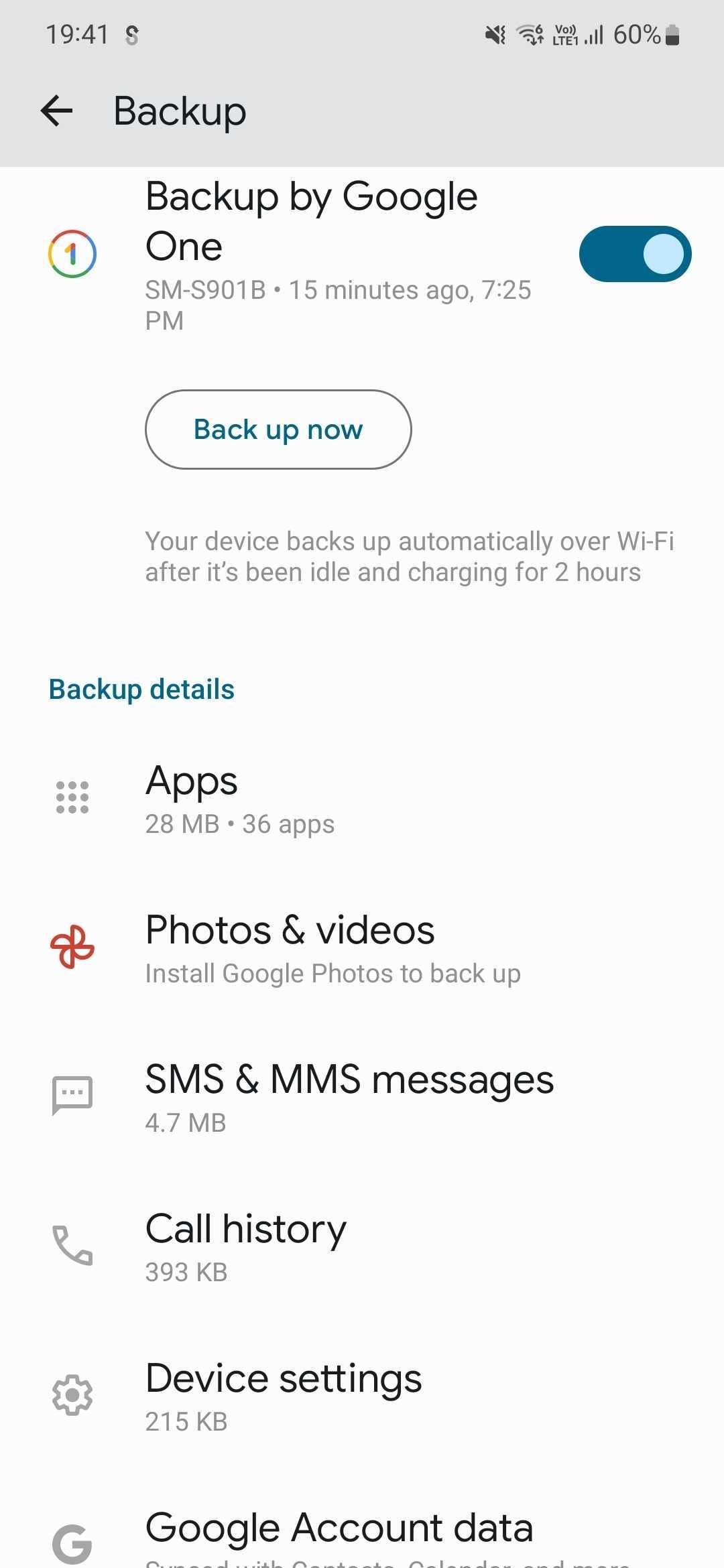**Category: Websites**

The image displays a phone screen with the time shown as 19:41 (7:41 PM). The phone is on silent mode, has a 60% battery life, and Wi-Fi is not enabled. The screen is part of a backup settings page.

At the top of the screen, there’s an option labeled "Backup" with an accompanying back arrow, allowing the user to exit this page. Below that, the text "Backup by Google One" is displayed next to the Google One logo, which is a multi-colored circle with the number "1" in the middle. The backup service is currently active, indicated by a switch turned on.

A button labeled "Back up now" is also visible. The status indicates that the last backup was performed 15 minutes ago at 7:25 PM, which intriguingly does not match the current clock time of 19:41. The screen notes that the device will automatically back up over Wi-Fi after it has been idle and charging for two hours.

The backup details listed include:
- Apps
- Photos and videos
- SMS and MMS messages
- Call history
- Device settings
- Google account data

The list is truncated, so additional backup items, if any, are not visible in the image.